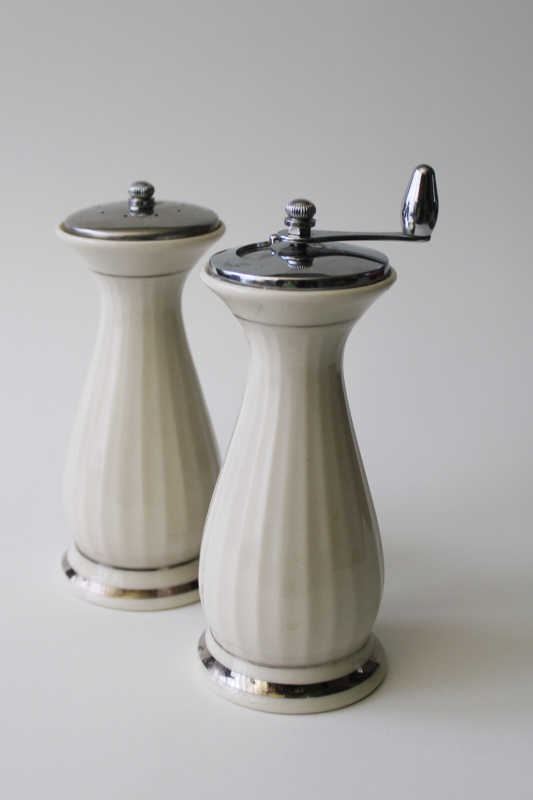The image features a pair of old-fashioned salt and pepper dispensers set against a gradient gray background, which transitions from dark gray in the upper right-hand corner to light gray in the lower left. The dispensers are creamy white, resembling a vase in shape—broad at the base, narrowing towards the top, and then flaring out slightly again. Both have distinctive silver caps. The salt dispenser, positioned slightly in the background, has multiple small holes for dispensing salt. The pepper grinder in the foreground is topped with a metal lever that extends upwards and is used for grinding pepper. Each dispenser also features two metallic rings near the base—one thinner and positioned slightly above the other thicker ring at the bottom, adding to their vintage charm.